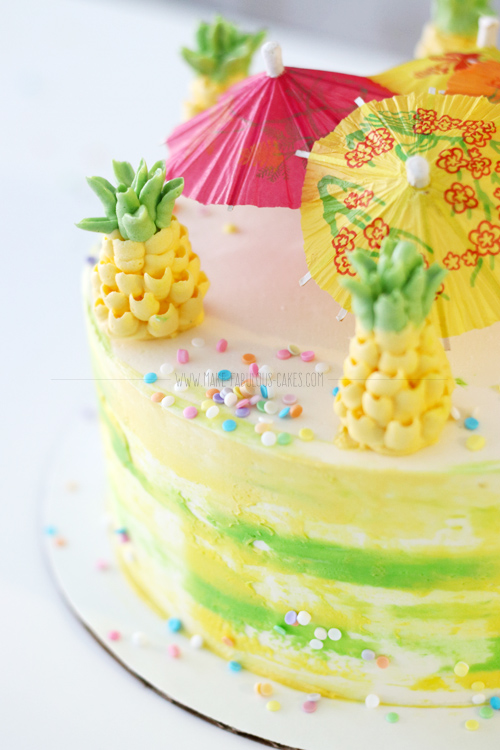This photograph captures a festive and intricately decorated cake, prominently featured on a white counter with a blurred background, ensuring all the focus remains on its vibrant details. The round, multi-layered cake, from the website makefabulouscakes.com, showcases a primary white frosting base adorned with sparkly candy pieces and light pastel-colored sprinkles distributed across the surface. Encircling the top are four ornate, frosting pineapples at intervals resembling a clock's positions, created with yellow frosting and green 'leaves.' Stabbed into the center are three cocktail umbrellas in yellow, orange, and red, enhancing the tropical, Hawaiian, or tiki bar aesthetic. This celebratory cake exudes a whimsical, tropical vibe, ideal for any festive occasion.